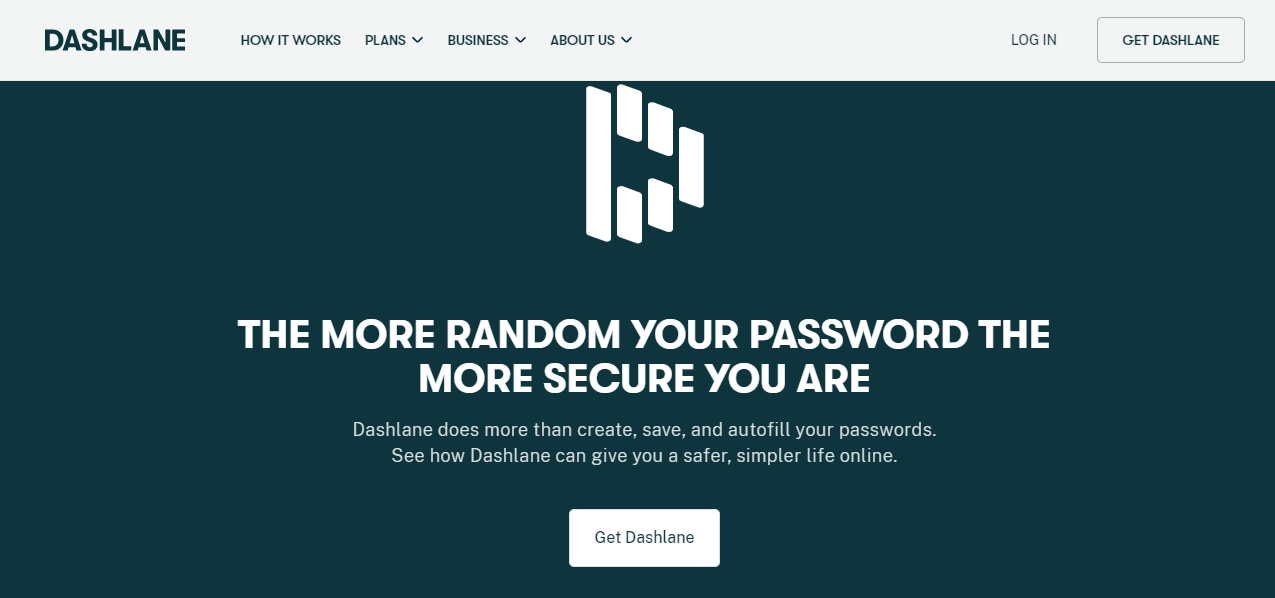A screenshot of the Dashlane website home page, featuring a sleek design primarily in dark blue and white. The top navigation menu includes categories such as "How It Works," "Plans," "Business" with a dropdown menu, "About Us" with a dropdown menu, "Plans" with a dropdown menu, "Login," and a prominent "Get Dashlane" button. The main message on the page highlights Dashlane's capabilities beyond just creating, saving, and autofilling passwords, suggesting that using more random passwords increases security. The website emphasizes that Dashlane can provide a safer and simpler online experience. Despite the minimalist detail, the overall theme conveys trust and simplicity through its color scheme and straightforward layout.